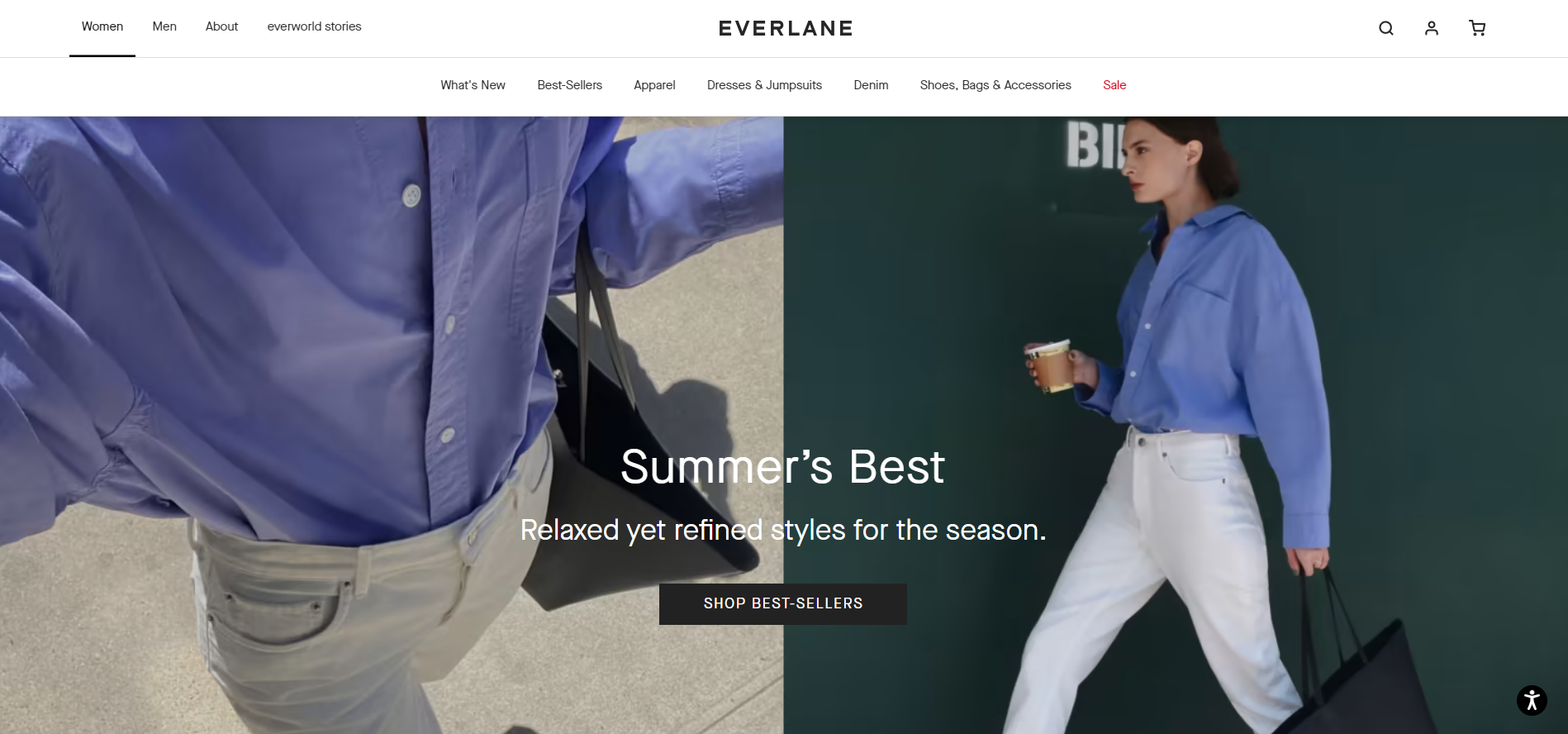The screenshot captures the homepage of Everlane, a fashion retailer. The header is minimalist with a plain white background showcasing the navigational menu. Centrally aligned, the word "EVERLANE" is prominently displayed in black, uppercase font. The menu options below are arranged from left to right as follows: What's New, Best Sellers, Apparel, Dresses & Jumpsuits, Denim, Shoes, Bags & Accessories. The final option, "Sale," is highlighted in red.

Beneath the navigation bar, two large photographs dominate the screen. The left image features a close-up of a woman's torso adorned in a blue button-down shirt paired with extremely faded skinny jeans. The right photograph displays a side profile of another woman against a greenish-gray background. The woman, a white brunette, is in motion, wearing a purplish-blue shirt and white skinny jeans. She holds a tote bag in her left hand, extending out of the frame.